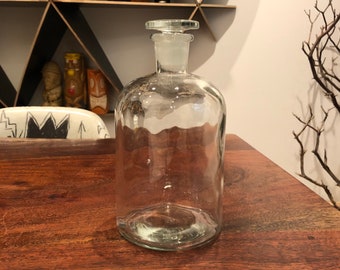This detailed photograph features a clear glass jug, centrally positioned on a dark reddish-brown wooden table. The jug has a wide, cylindrical body, gently curving into a rounded shoulder and a narrow neck, capped with a distinctive flat glass stopper that becomes milky white near its base. This stopper is firmly nestled in the neck, suggesting the jug is either empty or filled with a clear liquid like water.

The background is richly detailed; behind the jug, the upper edge of a white chair with a three-pronged, crown-like design filled in with black can be seen, giving the chair an ornate, jagged zigzag appearance. To the right, branches or driftwood, possibly part of a grapevine, extend into the frame, adding a natural element to the composition. Hanging above the chair on the left side of the image are three books positioned on triangular shelves built into the wall, contributing to a sense of organized eclecticism.

Additionally, there’s a suggestion of a maritime theme, with a rowboat or canoe displayed upright in the distant background, possibly part of a larger exhibition. The table's medium-brown wooden surface, visible knots, and texture add a grounded, rustic charm to the setting. Overall, the photograph captures a harmonious blend of natural elements and carefully curated objects, centered around the elegantly designed glass jug.